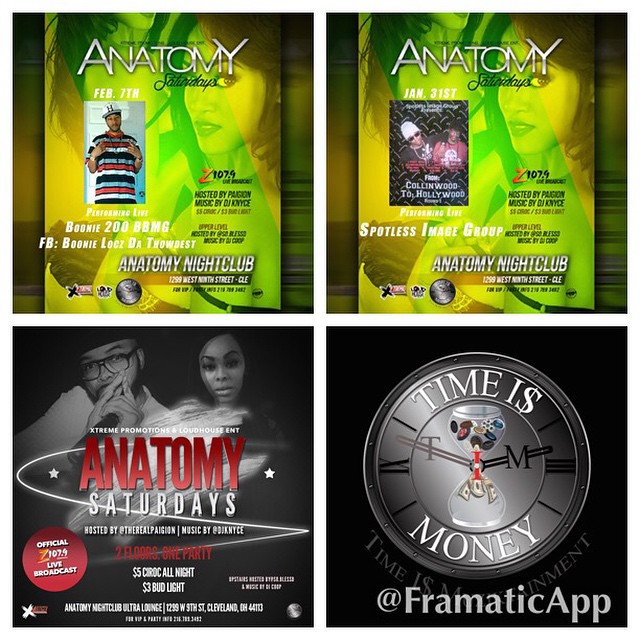The image is a promotional ad for "Anatomy Saturdays" at a nightclub, divided into four quadrants by a white line. In the top left quadrant, there's a green promotional flyer for an event on February 7th, featuring a young black man wearing a white cap and a striped shirt in black, red, white, and gray. Text on the flyer reads "Performing Live: Booney 200, BBMG, FB, Booney Locks, Throw Dust." The background includes images of women in lingerie.

The top right quadrant showcases another green flyer, this one for an event on January 31st. It features a graphic of two black men with the headline "From Collinwood to Hollywood" and states "Presenting Live: Spotless Image Group."

The bottom left quadrant contains a black-and-white image featuring a black man in a black hat, beard, and glasses beside a black woman. The overlying text reads "Anatomy Saturdays," with "Anatomy" in red and "Saturdays" in white. This section also includes the text "Official Z107.9 Live Broadcast."

In the bottom right quadrant, there is a silver clock with an hourglass in the center, filled with money and poker chips instead of sand. Around the dial, it reads "Time is Money," and the text below states "at Phramatic App" in gray.